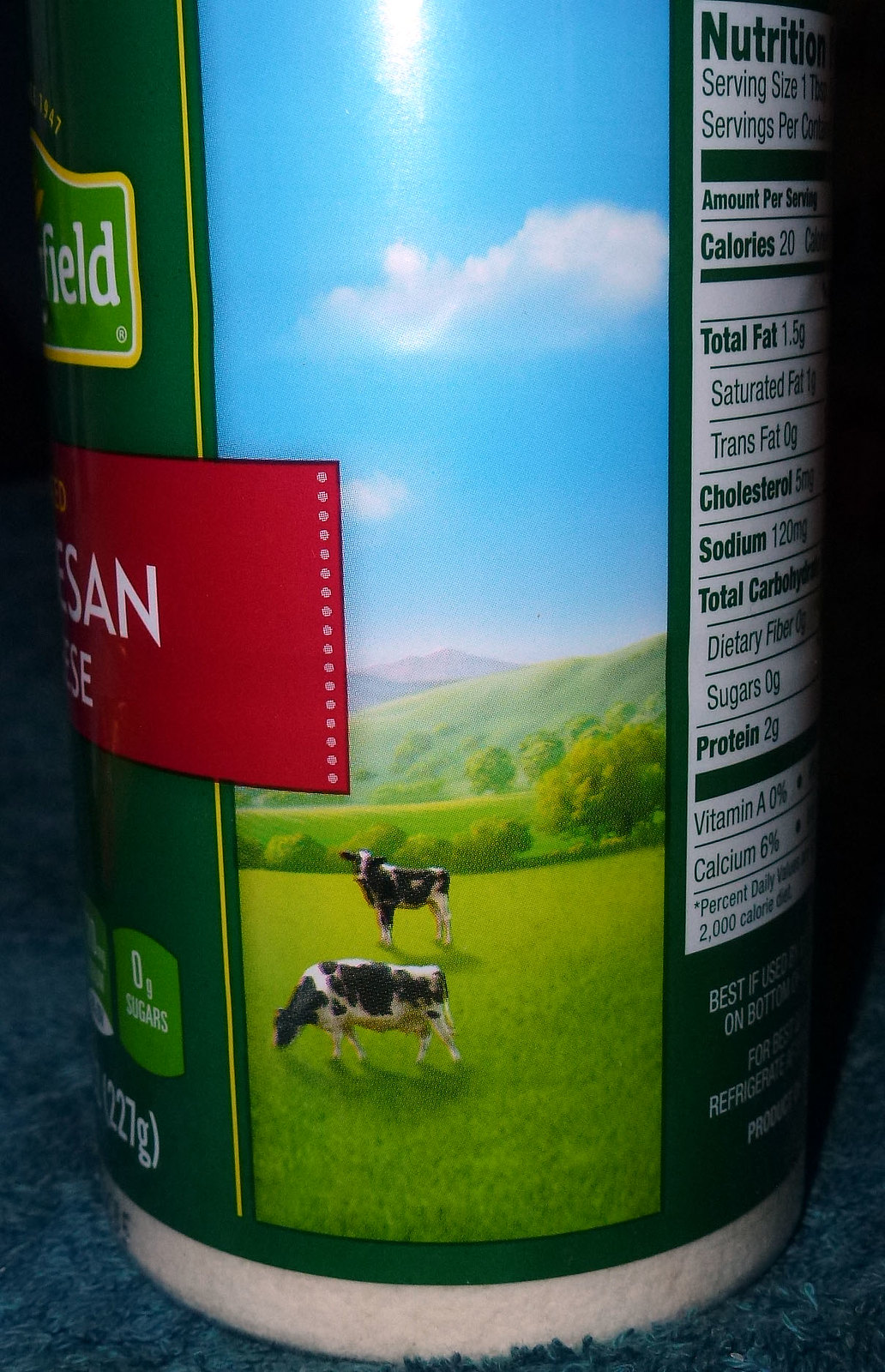This is a detailed close-up photograph of a cylindrical, round plastic container of shredded Parmesan cheese. The container features a green label that wraps all the way around it, with a little red banner across the front displaying the words "Parmesan cheese." Towards the top of the container, there's a partially visible brand name, ending in "field." The label also includes a prominent note indicating "zero grams of sugars" in a green square.

Dominating the front of the container is a picturesque image of a meadow under a bright, sunny day. The scene includes two black-and-white cows; one cow is grazing while the other stands and gazes into the distance. The meadow has a mix of light and dark green grass, with light green fields and flowing hills flanked by darker green areas. In the backdrop, there are round-topped, light green trees, and further still, a gray mountain ridge. The sky above is a vibrant cyan blue, accentuated by wispy white clouds with darker blue undersides, and a cascade of light creating a white splotch on the image. The photograph on the container evokes a clear, daytime ambiance.